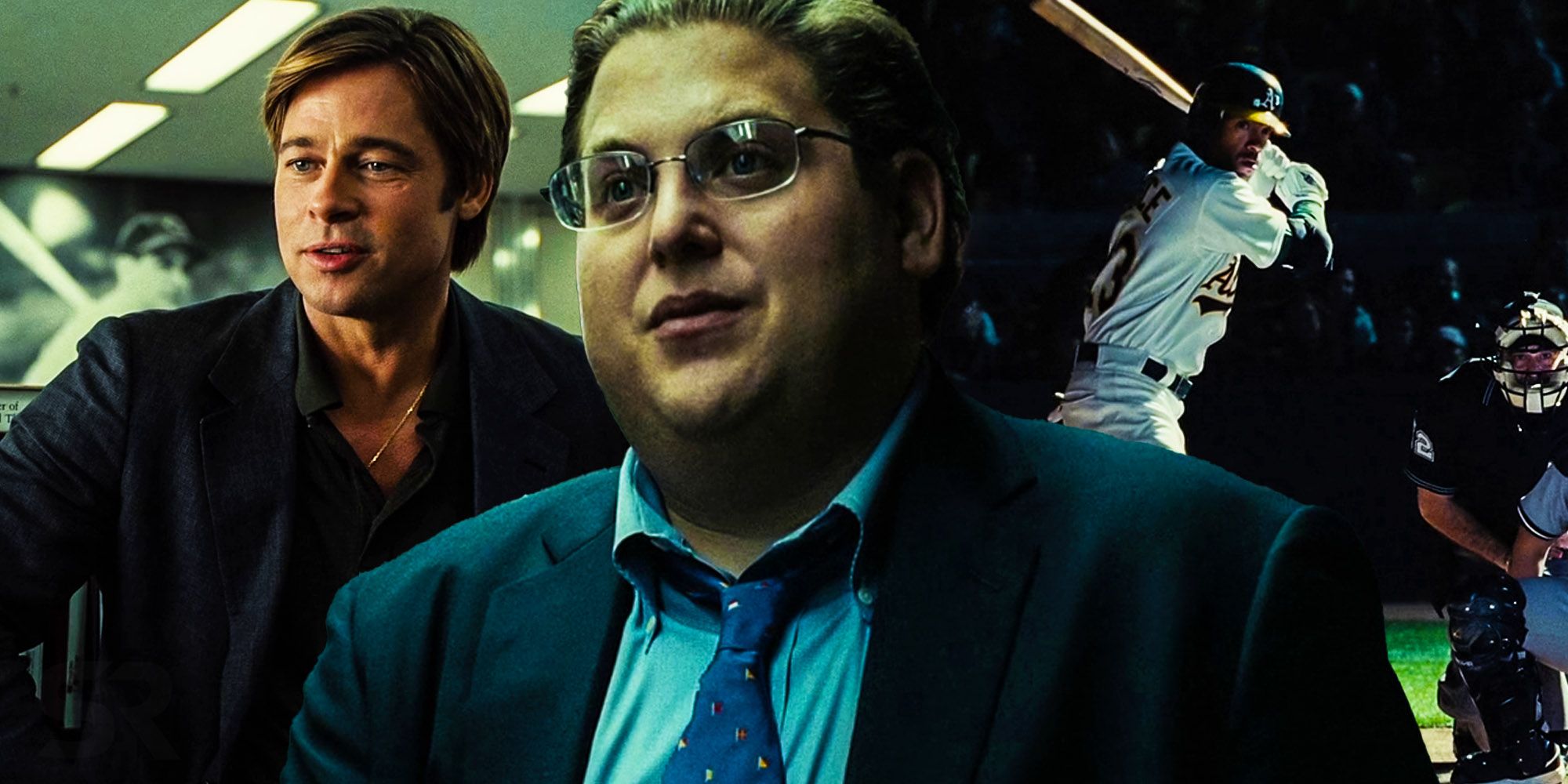This detailed descriptive caption synthesizes information from all the given descriptions:

This image is a scene from the movie Moneyball, featuring two distinct elements. In the forefront on the left, Brad Pitt and another actor stand side by side, both wearing suits. The unidentified actor, slightly overweight and wearing a blue suit with a light blue shirt and blue tie, also has glasses and is looking intently at something off-screen. Brad Pitt, with longer hair and a gold chain around his neck, is similarly focused on the same spot. On the right, in the background, a baseball game unfolds. A player in a white uniform, whose team cannot be identified, is poised to swing his bat. Behind him, a catcher wearing a traditional mask and a short-sleeved dark blue jersey is squatting, seemingly conversing with another player. The overall image is dark and muted, capturing the serious mood and tense atmosphere of the scene.